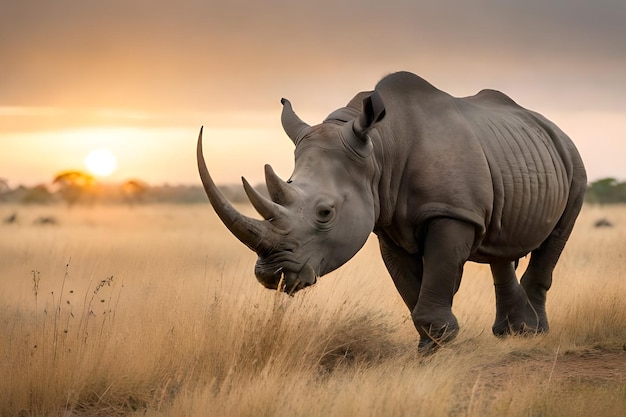In this captivating photograph taken during a safari, a majestic rhinoceros is captured mid-stride in a natural, sunlit setting. The powerful beast, with its velvety gray, almost brown skin, dominates the right-hand side of the frame. Its distinct three horns are prominently showcased – with a long, curved primary horn at the front and two smaller ones trailing behind on its head. The rhino's pointed, rounded ears add to its grandeur.

In the background, a bright beige grass savanna stretches out, blurred slightly by the camera, giving depth to the setting. A thin, dark gray strip of silhouetted forest lines the horizon, punctuated by the characteristic arched shapes of acacia trees. On the far left, the sun sets in a brilliant display, appearing as a white ball with a glowing orange halo. The sky transitions from a beige to yellow hue near the horizon, encircling the sun, to a thick band of gray clouds with brown highlights above. This detailed backdrop enhances the serene yet wild beauty of the scene, emphasizing the inherent tranquility and raw power of the rhinoceros in its natural habitat.